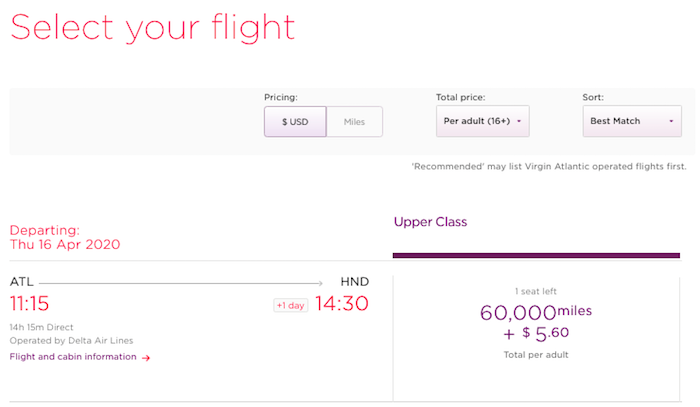A detailed descriptive caption:

The interface of a travel booking or airline site prominently features Virgin Atlantic flights, with the main section inviting users to "Select Your Flight" in pink text at the top left corner. Currency options are provided, displaying prices in US Dollars (USD) alongside an option to select mileage points for the flight cost; the USD option is currently selected. The total price per adult, defined as individuals aged 16 and older, is shown underneath.

Users can sort flight options by various criteria such as "Best Match" and "Recommended," with Virgin Atlantic flights appearing prominently in the listings. A specific flight details section indicates that the departure is scheduled for Thursday, 16th April 2020. The route is from Atlanta (ATL) to Haneda (HND) airport. Departure from Atlanta is at 11:15 AM, and the arrival time at HND is 2:30 PM on the following day (plus one day), with a total flight duration of 14 hours and 15 minutes. This direct flight is operated by Delta Airlines. All relevant times and dates are displayed in pink text.

Additional flight and cabin information can be accessed via a purple text link with a pink arrow to the right. A long gray arrow visually connects the two airports’ names.

Adjacent to this information, an "Upper Class" section is highlighted in purple. Below a dark purple bar, it is noted that there is only "One Seat Left." The cost for this seat is 60,000 miles plus $5.60, displayed in purple text. The "Total Per Adult" price is shown in gray text immediately below this.